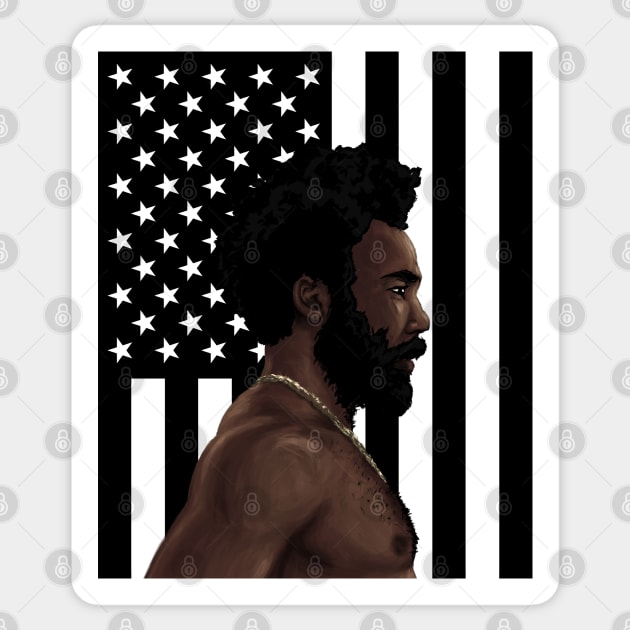The image is a stylized clipart of an African-American man, likely Donald Glover, depicted in an animated, cel-shaded style. He is shown from the chest up, facing to the right, with big, fluffy hair and a full, bushy beard. He is shirtless and adorned with a gold chain around his neck. His expression is neutral. Behind him, a black and white American flag is oriented vertically, adding a contrasting backdrop. The entire image is overlaid with numerous watermarks resembling small padlocks, contributing to the clipart feel.